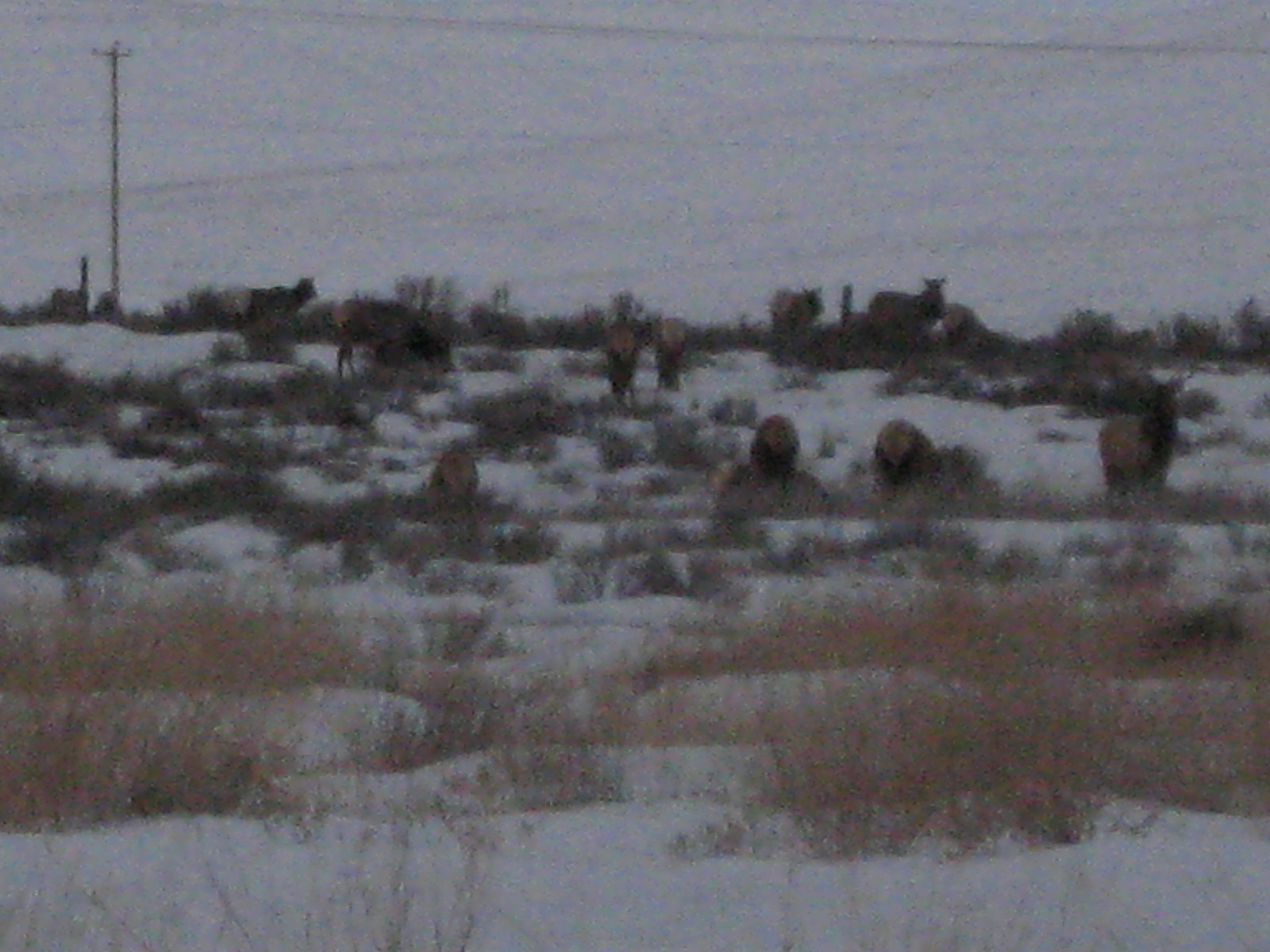The photograph is a grainy, low-light image capturing a gray, wintry day in the countryside. The ground is blanketed in white snow, with patches of brown dead grass and weeds poking through the surface. In the foreground, a series of bristly, light brown bushes add texture to the snowy landscape. Toward the right of the image, an indistinct animal figure appears to have antlers, although the blurriness makes it hard to confirm. Further back, a number of large, dark brown livestock animals—either cows or horses—graze among the snow-covered patches of grass. The horizon is lined with a series of muted trees, and a tall telephone pole stands prominently in the background, with an accompanying telephone wire stretching across the scene. The photograph has a muted, monochromatic palette and a grainy texture, suggesting it was taken on film.